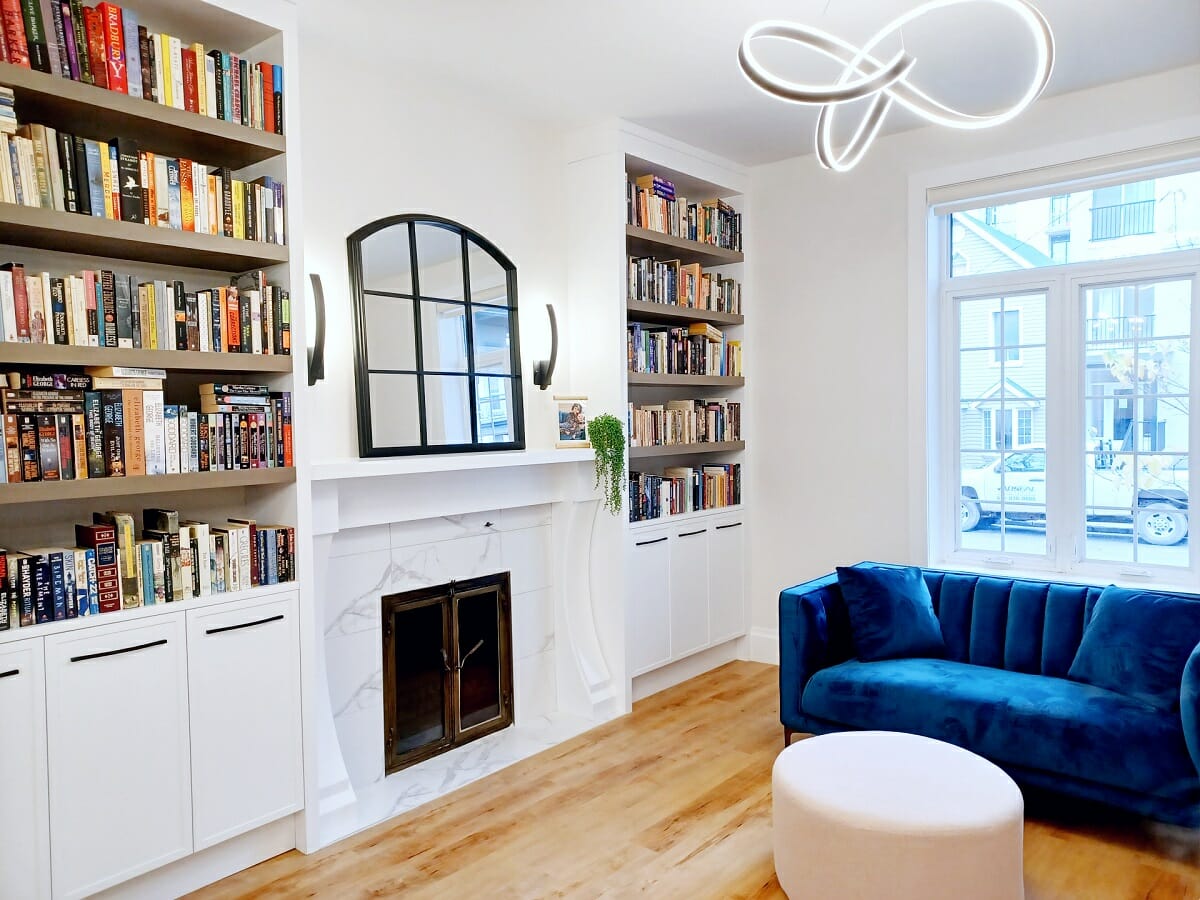The image captures a stylish and comfortable living room that evokes an air of modern elegance. The room's focal point is a white marble fireplace with a glass door and brass or bronze accents, crowned by a large arched mirror. On either side of the fireplace are tall, built-in bookshelves that descend two-thirds of the way down the wall, transitioning into paneled cabinets with black handles. The bookshelves, which are filled with a variety of books, feature five fully stocked shelves, lending a cozy library feel to the space.

A striking feature of the room is the vibrant blue velvet couch, adorned with two matching blue pillows at each corner. In front of the couch sits a white circular ottoman, offering a comfortable spot to rest your feet. The room's wooden floors are a light, almost blonde, wood that complements the overall white color scheme, including the white walls that maintain a clean and airy ambiance.

Adding to the modern aesthetic is a unique, twisted light fixture that loops gracefully in the center of the room. To the right of the couch, a large double window with white trim opens up the space, offering a view of a street where a truck and another house can be seen. A small plant cascading over the mantel and a framed photograph contribute subtle yet personal touches. On either side of the mirror above the fireplace, elegant wall sconces enhance the room’s sophisticated look, rounding out a space that is as inviting for reading and relaxation as it is for modern living.